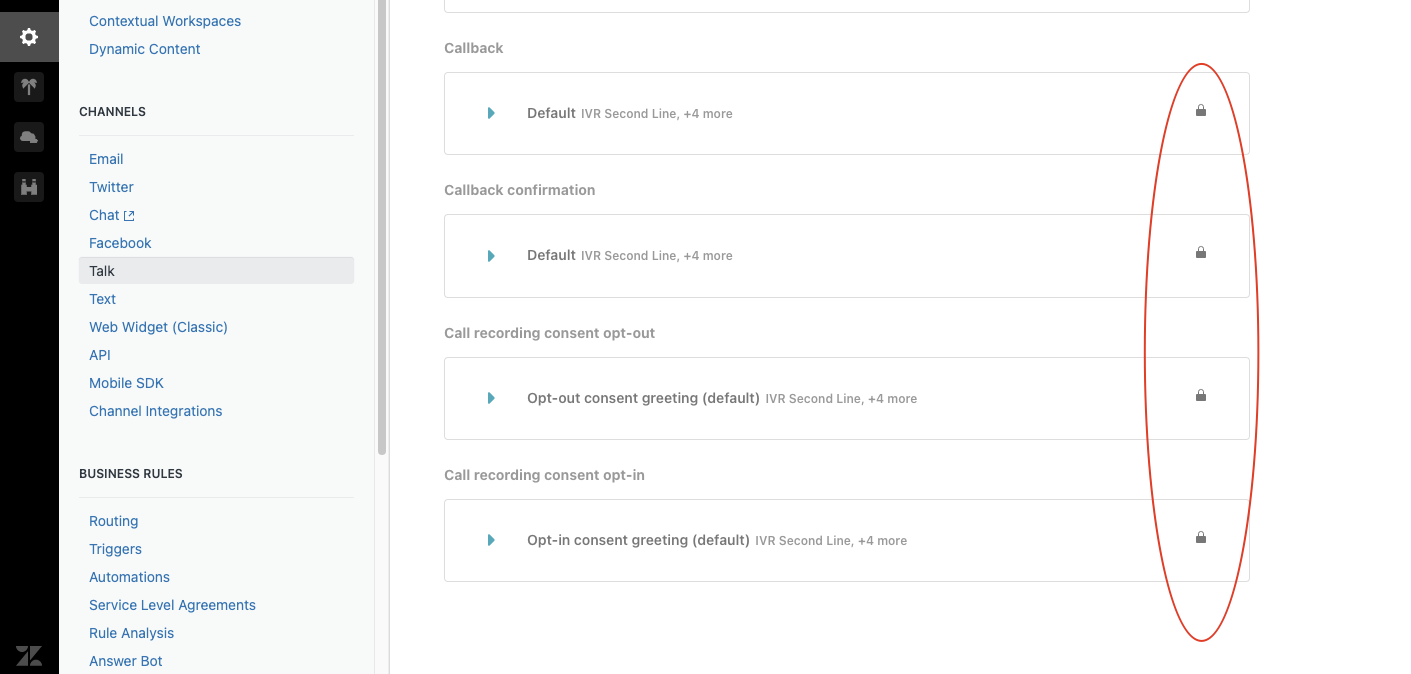The image on the left features a black column with headings that include "System," "Signal," and "Storage." Below these, there are icons depicting two individuals. To the right of this black column, in blue text, it reads "Contextual Workplaces" and "Dynamic Content." Parallel to this, in black text, is the heading "Channels," beneath which are listed several communication platforms: "Email," "Twitter," "Chat," "Facebook," and "Talk," with the "Talk" option highlighted in gray.

Below these channels are additional options including "Text," "Wedge Widget," "Classic," "API," "Mobile SDK," and "Channel Integrations." Following this, various business process features are listed: "Business Rules," "Routing," "Triggers," "Automation," "Service Level Agreements," "Rule Analysis," and "Answer Bot."

Further right, the image includes the term "Callback," followed by a right arrow and the text "Default IVR Second Line" plus "Four More." This is repeated with variations for different functionalities: "Callback Confirmation," "Call Recording," "Consent Opt-Out," "Consent Greeting," and "Call Recording Consent." Each of these is accompanied by the notation "Default IVR Second Line plus four more," indicating additional, unspecified options.